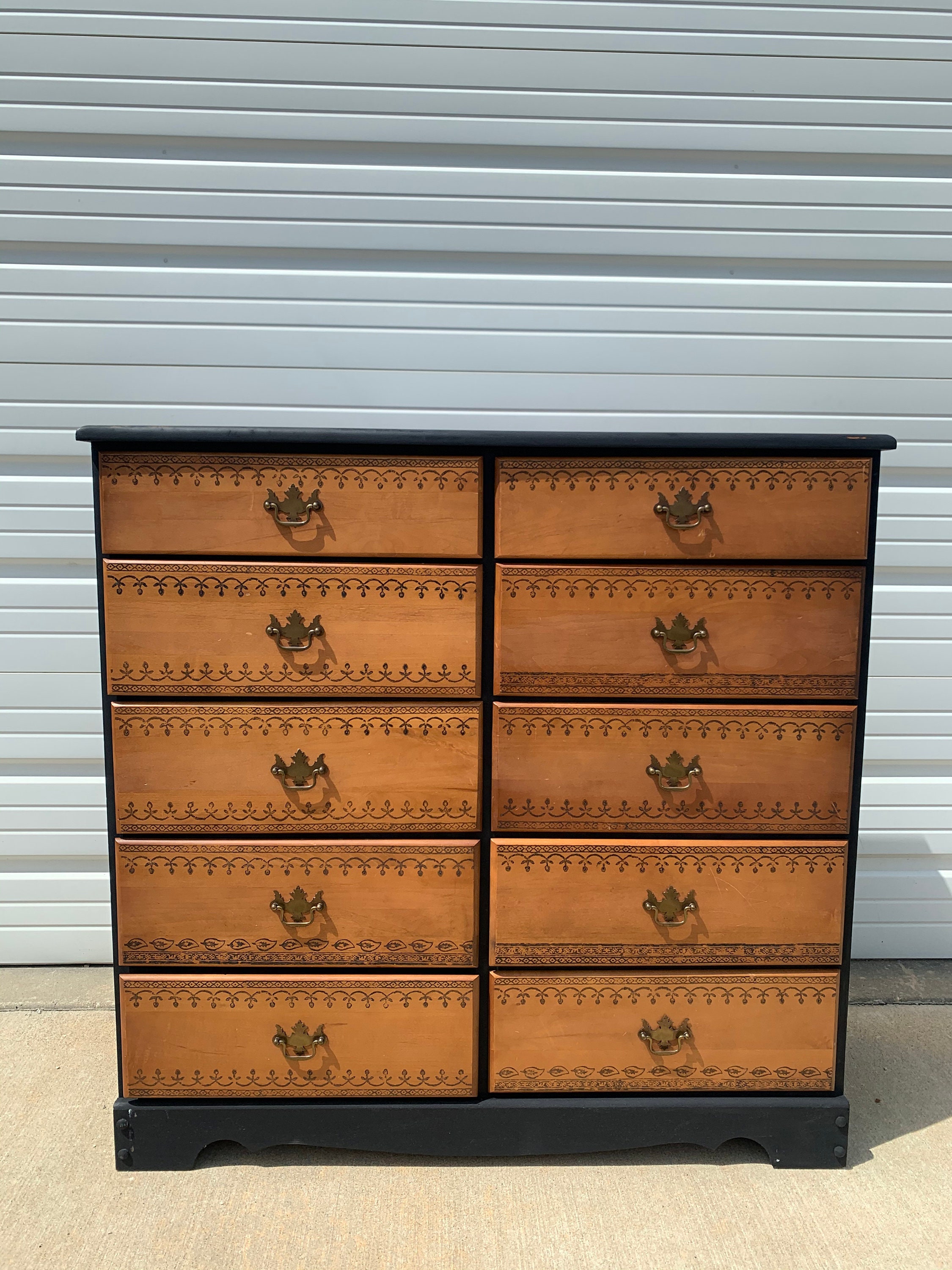The image is a clear, detailed photograph of a wooden dresser placed outdoors, as evidenced by the bright, natural lighting and harsh sunlight casting strong shadows. The background features a light gray garage-like door, suggesting the setting is in front of a panel or storage unit door. The dresser is a square piece, divided into two vertical sections, each containing five neatly stacked drawers, making a total of ten drawers. The base and the top surface of the dresser are black, while the drawer fronts are a natural wood color adorned with decorative patterns. Each drawer is equipped with a centrally positioned handle made of a gold-tinted metallic material. The photographer captured the dresser directly from a frontal viewpoint, suggesting a focus on the dresser's details and symmetry. The presence of a variety of colors—light brown, black, gray, and tan—adds to the visual interest of the image.